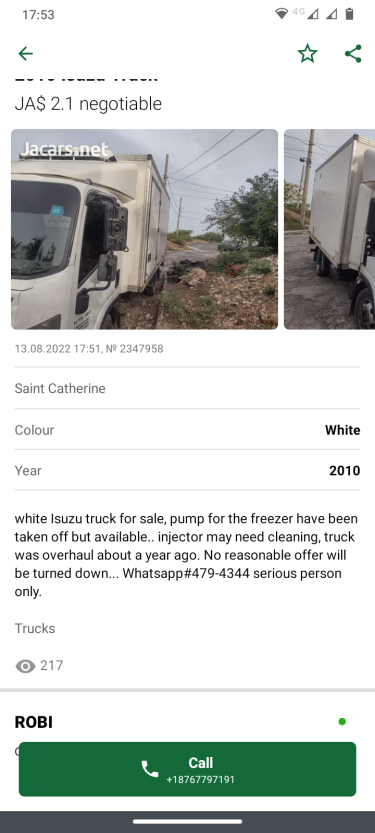Screenshot of a buy-and-trade platform (either a website or app) features a layout with icons indicating the time (17:53 or 5:53 PM), Wi-Fi connectivity, 4G signal strength, and battery life at the top. Below these icons, the page displays a listing for a vehicle:

**Listing Title:**
JA - White Isuzu Box Truck For Sale

**Details:**
- **Price:** 2.1 (Negotiable)
- **Location:** St. Catherine
- **Color:** White
- **Year:** 2010
- **Description:** A white Isuzu truck available for purchase. The truck is equipped with a freezer, though the pump for the freezer has been removed. The injectors may require cleaning. The truck underwent an overhaul approximately a year ago. The seller is open to reasonable offers.
- **Contact Information:** Interested buyers can reach out via WhatsApp at 479-434-XXXX for serious inquiries only.

**Category:** Trucks
**Total Listings:** 217

At the bottom of the listing, there's a prominent green "Call" button for direct contact with the seller.